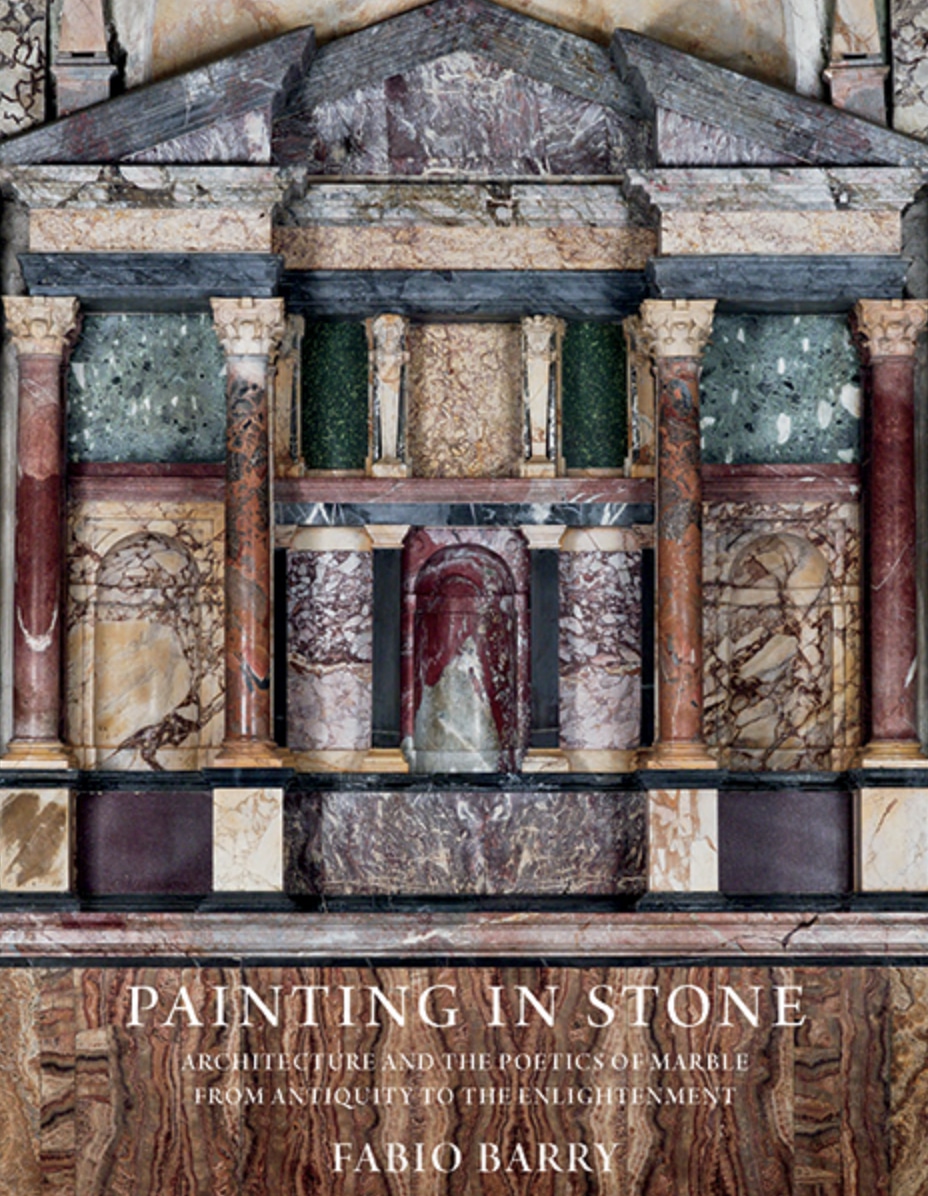The book cover prominently features an intricate formation of stones, meticulously arranged to resemble an architectural structure. The top section showcases an arched roof created by gray rocks, many of which are artfully split in half and meet at the arch's apex. Below this, the stone arrangement transitions into various sections of color: gray, light yellow, and dark gray rocks, portraying a ceiling-like division. Descending from this point are four columns, each adorned in a palette of brown and light orange, interlaced with webs of blue, adding intricate details to the façade. Towards the bottom, in white lettering, the title reads, "Painting in Stone: Architecture and the Poetics of Marble from Antiquity to the Enlightenment" by Fabio Barry. The overall appearance of the stones emphasizes a variety of natural hues, including browns, reds, greens, and grays, some solidly colored and others intricately designed, reflecting a poetic interplay of color and form in the depiction of this stone structure.